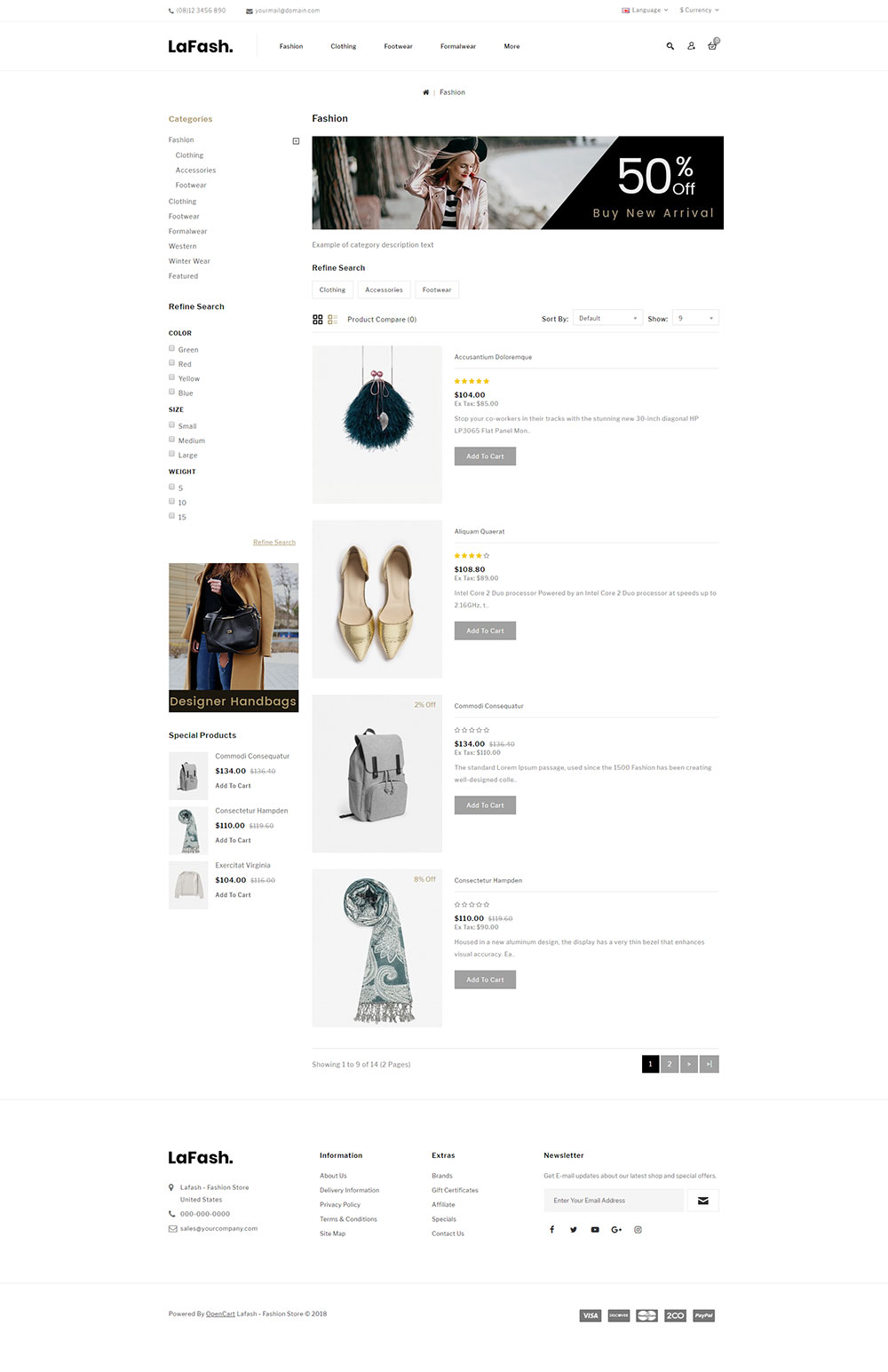The image showcases a webpage from "LeFache," a designer accessory store. On the top left of the page, the brand name "LeFache" is prominently displayed. The website appears to specialize in various accessories, including bags, scarves, shoes, and purses, targeted towards fashion-forward customers. 

The top navigation bar features multiple categories such as "Fashion" and "Catalog," among others, for easy browsing. A striking image of a woman is displayed with a promotional text beside her offering "50% off" on new arrivals. Below this, the term "Fashion" is mentioned again, reinforcing the site's focus. 

Highlighted across the webpage are at least four distinct items: a fluffy blue accessory with a five-star rating, a pair of goldish-yellow high heels rated with four stars, a gray backpack, and a bluish scarf. To the left of these items, an image of another woman in a brown jacket holding a designer handbag is visible, accompanied by the text "Designer Handbags."

On the left sidebar, filters to refine the search by color and possibly other attributes are available. At the bottom of the page, there are additional links to various sections of the site for further exploration.